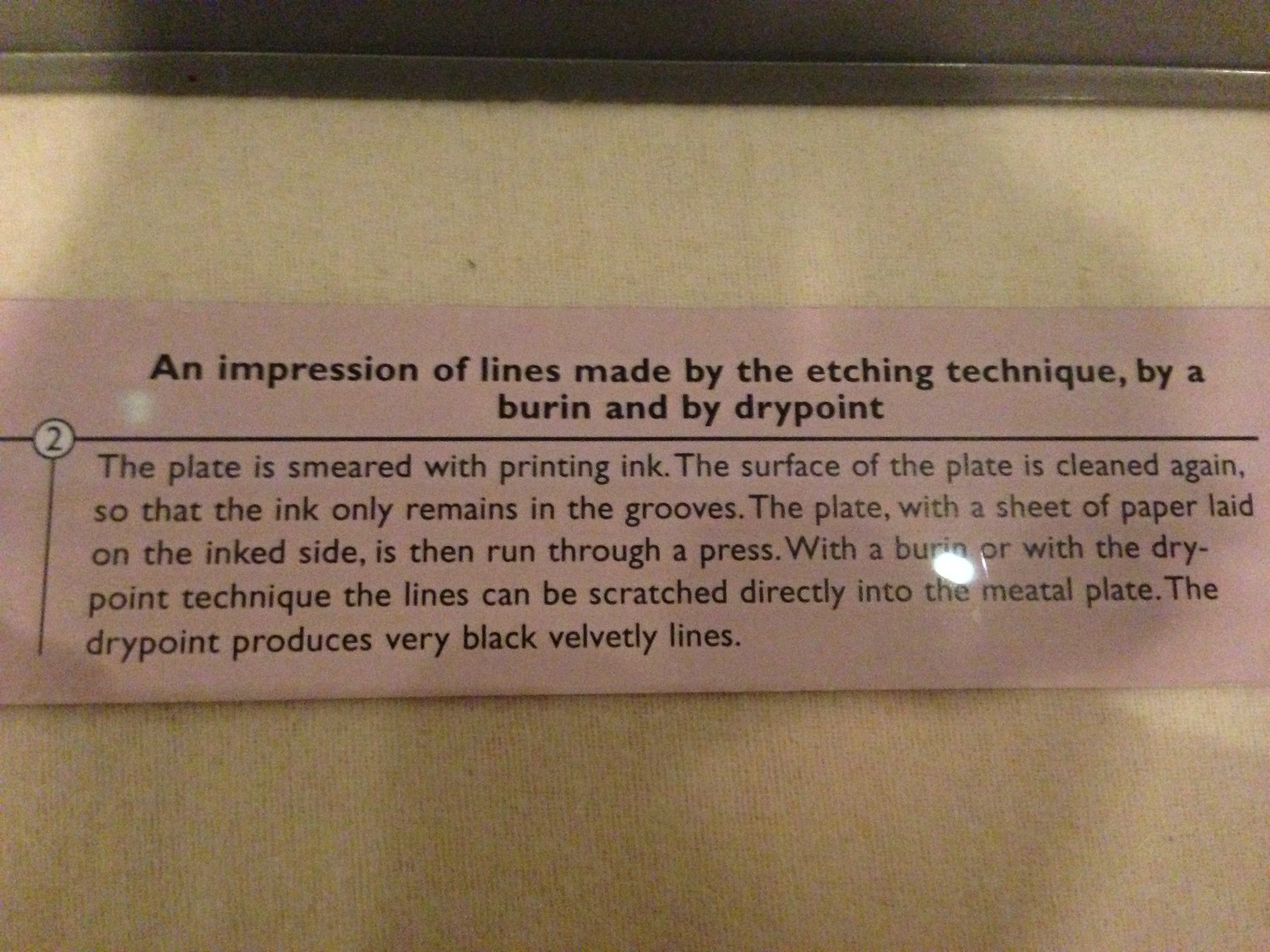The image depicts a descriptive placard, potentially observed in a museum setting, against a textured light tan background. The rectangular pink piece of paper is bordered by a thin, dark brown and black frame, contributing to the polished appearance under the reflective glass cover. 

At the top of the paper, bold black text reads: "An impression of lines made by the etching technique, by a burin and by drypoint." Below a separating black horizontal line, there's a black-bordered white circle containing the number "2" at the intersection of two lines—one running horizontally and the other vertically downward.

The subsequent detailed explanation, written in thinner black text, states: "The plate is smeared with printing ink. The surface of the plate is cleaned again, so that the ink only remains in the grooves. The plate with the sheet of paper laid on the inked side is then run through a press. With a burin or with the drypoint technique, the lines can be scratched directly into the metal plate." A noted typo appears in this section, spelling "metal" as "m-e-a-t-a-l." The concluding sentence notes, "The drypoint produces very black, velvety lines."